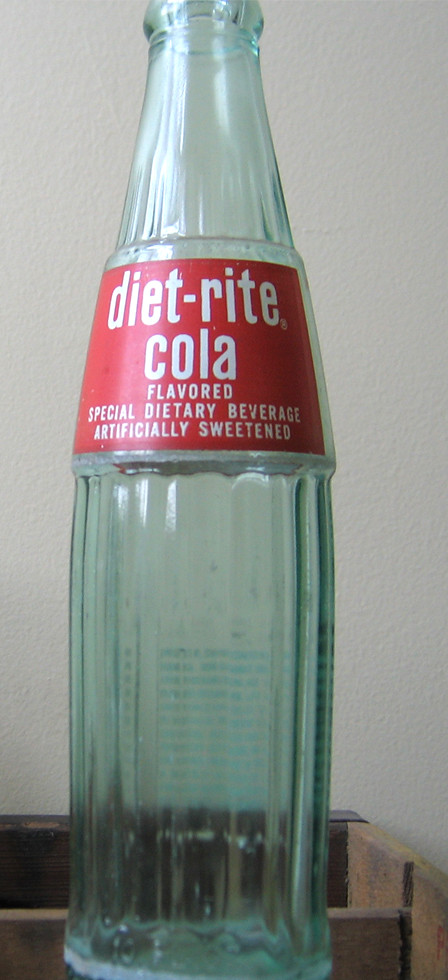The image depicts an up-close photograph of an old-fashioned, empty glass soda bottle made from thick bluish-green glass, taking up nearly the entire frame. The top part of the bottle is slightly cut off, revealing only the first half of the slender bottleneck. The bottle, with numerous ridges, tapers from its wide base towards the neck. Prominently displayed in the middle of the bottle is a red label with white lowercase writing. This label reads: "diet rite cola," centered in three lines, with additional text below stating "flavored special dietary beverage, artificially sweetened." The clear backdrop features an off-white wall, while the bottle itself rests on a wooden shelf or table with a visible edge on the right-hand side. The detailed glass texture and ridges of the bottle are clearly visible, adding to the vintage aesthetic of the image.